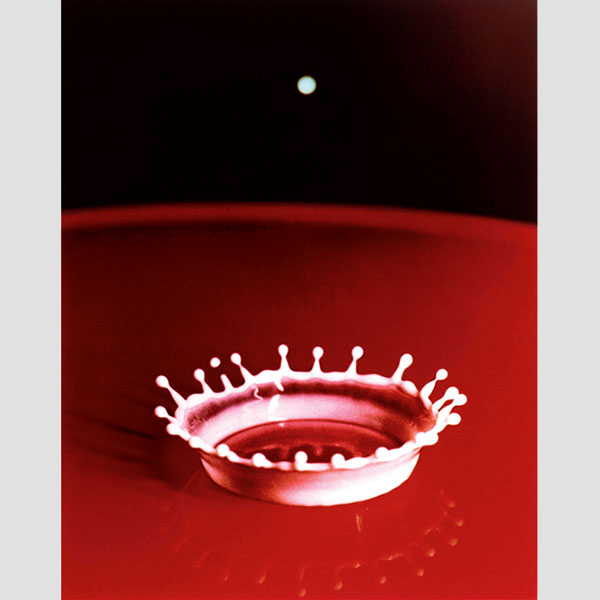This vertically aligned rectangular image, framed by thick light gray borders on the left and right sides, captures a striking splash phenomenon. The upper third of the image is a solid black expanse, punctuated only by a small, perfectly round white dot centrally positioned. Below this black expanse, the image transitions into a vibrant red liquid encompassing the lower two-thirds of the frame. 

At the heart of the red liquid, a striking white circular splash shape emerges, reminiscent of a corona, with red outlines accentuating its form and small drops radiating from its rim. This splash creates the illusion of a bowl with red at its base and white-tinted edges, intricately detailed with some red mixed in. The reflective quality of the surface beneath allows the edges of the splash to mirror, enhancing the complexity and depth of the visual.

Overall, the image features a stunning contrast between the minimalist black upper section and the dynamic red lower section, with the white splash acting as a focal point, symbolizing the moment of impact in liquid dynamics.